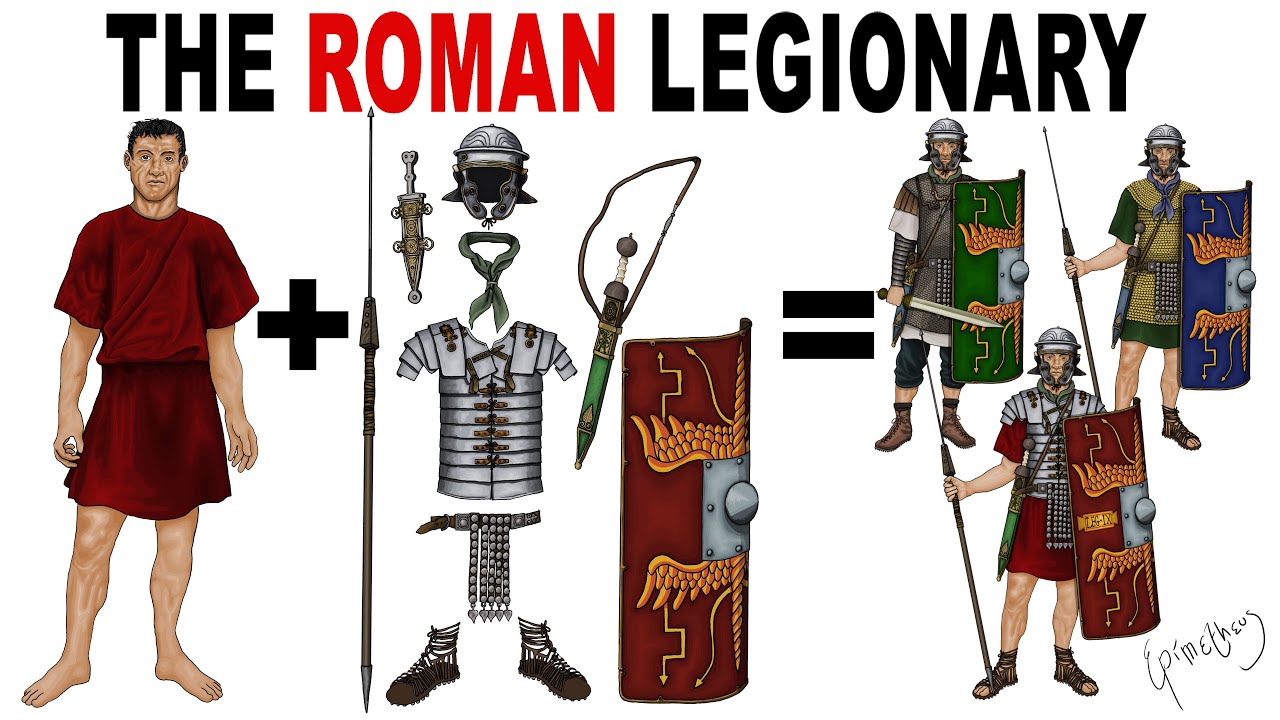The image is an illustrated guide against a white background detailing the attire of a Roman legionary, seemingly designed for a video game. At the top, bold text reads "The Roman Legionary," with "Roman" in red and the other words in black. On the left, there is an image of a man with short black hair, dressed in a red tunic and short skirt. Next to him is a large black plus sign, followed by a collection of Roman military gear: strappy sandals, a belt with a cod piece, chain mail armor, a neck scarf, the iconic Roman helmet with cheek guards, and a variety of weapons including a dagger, spear, long sword, and a red round shield. An equal sign to the right of this gear leads to three different fully equipped Roman legionaries, each holding different weapons and shields in different colors: one in a gray suit with a green shield, another in green armor with a blue shield, and a third in gray and red armor with a red shield. In the bottom right corner, the name "Epimetheus" is handwritten.